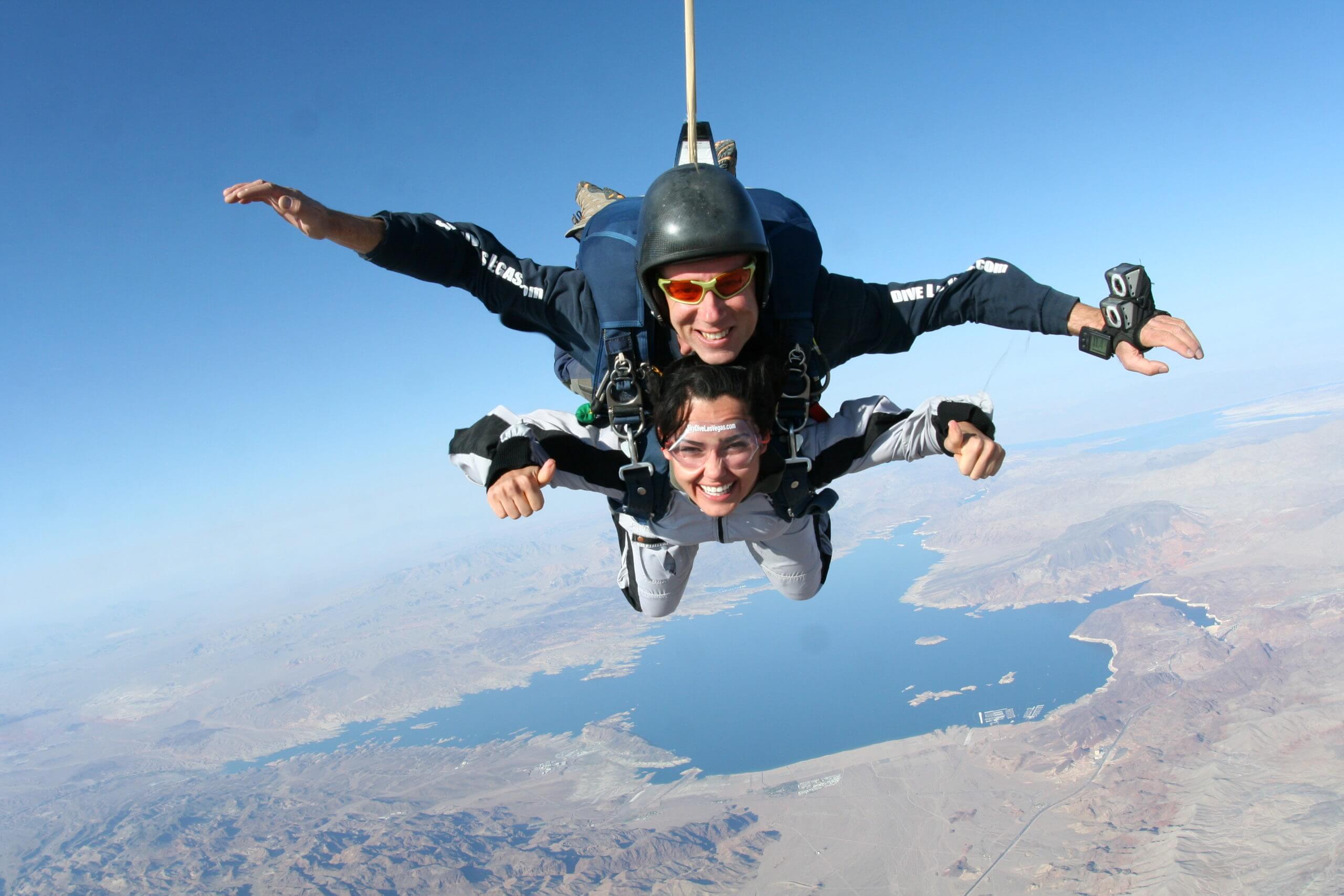The landscape image captures a thrilling moment of tandem skydiving, where a man and a woman are free-falling together beneath the clear blue sky. The male skydiver, likely the professional, is positioned on top with a rope and large parachute casing visible on his back. He sports a navy blue and black jumpsuit paired with a black helmet and pink goggles. Stretching his arms wide, he's smiling down at the camera, which is being operated by another skydiver. The woman, attached to the man, is dressed in a white outfit accented with black sleeves. Her short black hair flows freely as she extends her arms forward, giving enthusiastic thumbs up, and wearing clear goggles. Both skydivers are relishing the experience, with broad smiles on their faces. Below them, the earth's surface appears in a gray tone, dotted with patchy white clouds and featuring a large lake amidst what seems like a desert landscape, hinting at an altitude above 5,000 feet.